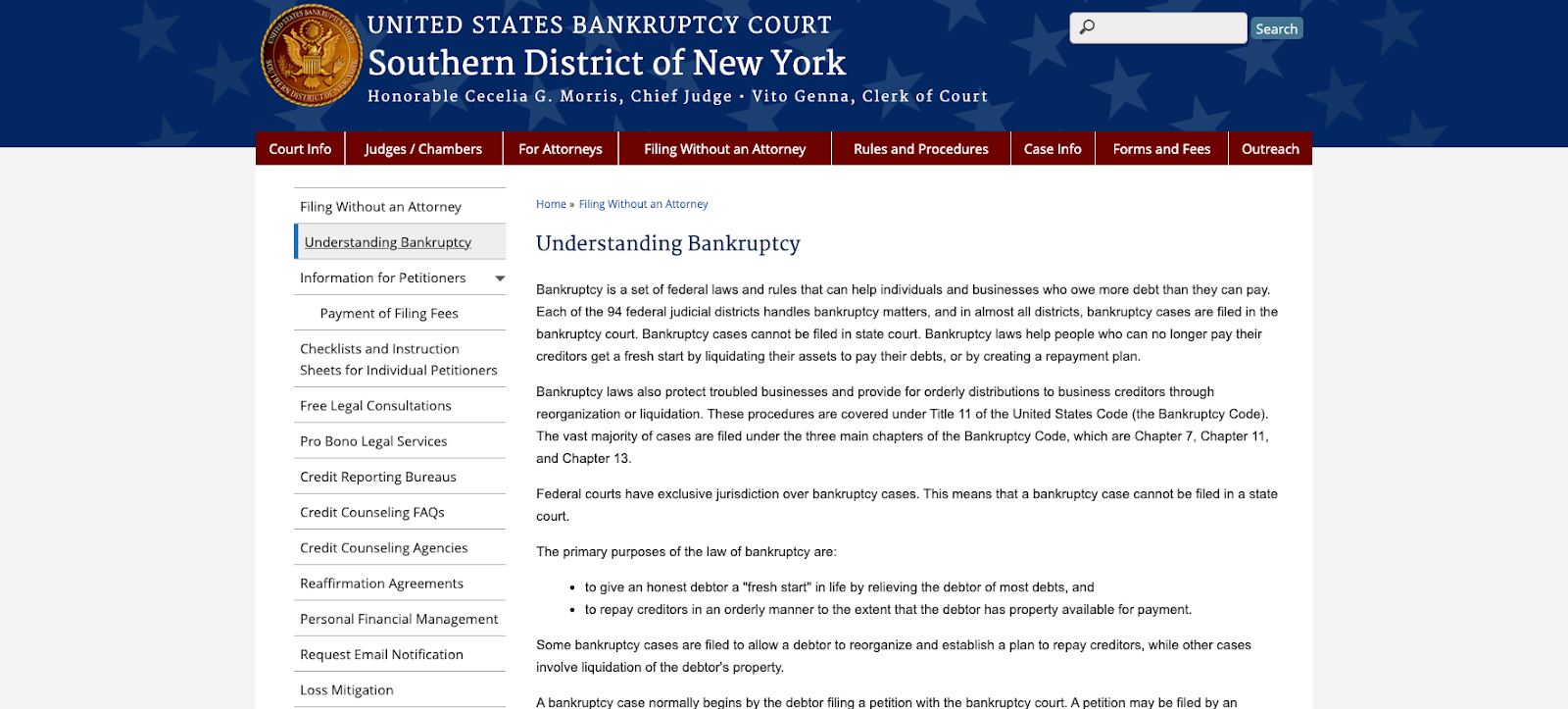**Image Caption:**

In the United States Bankruptcy Court for the Southern District of New York, the Honorable Cecilia Morris serves as Chief Judge, while Vito Gina holds the position of Clerk of Court. Their names are prominently displayed in a navy blue box adorned with stars and the court's seal.

The image explains the intricacies of bankruptcy, a set of federal laws and rules designed to assist individuals and businesses that are unable to pay off their debts. These laws provide two main solutions: liquidation of assets to settle debts or creation of a repayment plan. Managed exclusively by federal courts, bankruptcy cases are filed within the 94 federal judicial districts, with the Court overseeing most cases.

Bankruptcy laws, outlined in Title 11 of the United States Code, aim to give debtors a fresh start by relieving them of most debts and ensuring orderly repayment to creditors. These cases primarily fall under three chapters of the Bankruptcy Code: Chapter 7, Chapter 11, and Chapter 13. Whether helping a debtor reorganize their finances or liquidate their properties, bankruptcy ensures a systematic and fair process for all parties involved.